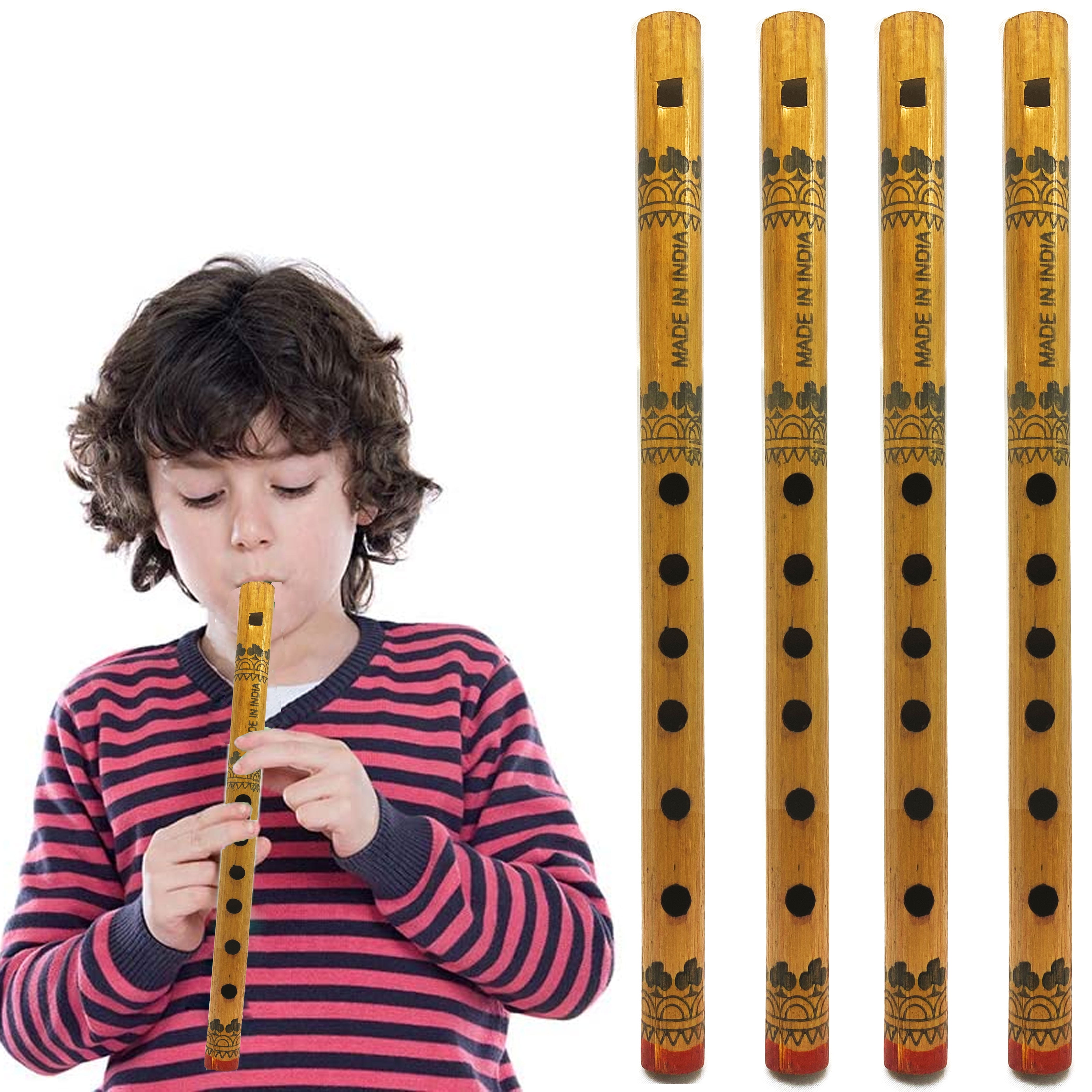The image features a Caucasian child with curly, shoulder-length, brown hair and long eyelashes, looking down as they blow into a wooden recorder-like instrument. The child, who has their eyes downcast, is dressed in a long-sleeved sweater with pink and blue stripes over a white shirt. The fingers on both hands cover some of the holes on the recorder, which has a total of six finger holes. 

On the right side of the image, there are four identical wooden recorders, showcasing their cylindrical shape, each adorned with a pattern of small tree decorations and circles. The instruments, marked "Made in India," have a square blowhole at the top followed by decorative patterns and the six unevenly spaced holes, ending with a distinctive red band. The background of the image is white, drawing clear attention to the child and the musical instruments.